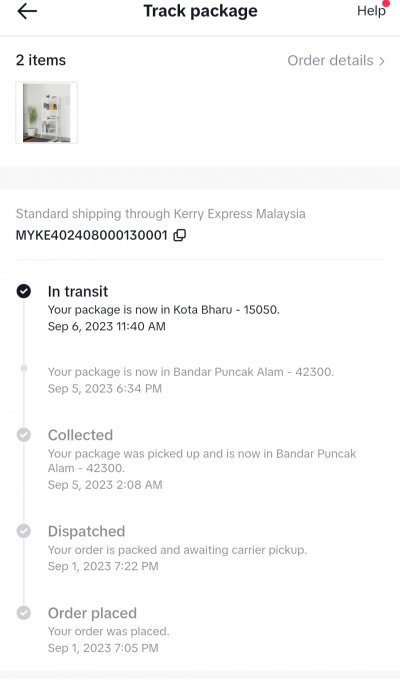On a white background, an interface is displayed showing tracking information for a package. At the top of the interface, there is a left-pointing arrow labeled "Track Package" and a "Help" option on the right. Directly beneath, aligned to the left, the text "Two items" is visible next to a small, blurry image whose contents are indiscernible. To the right of this image, the text "Order Details" is displayed.

Below this section, a grey area separates the header from the shipping details, which read as follows: "Standard shipping through Carey Express Malaysia, MYKE402-408000-130001." The current status indicates "In transit: Your package is now in Kota Bharu, 15050, on September 6th, 2023, at 11:40 AM." Previously, the package was noted to be "In transit: Your package is now in Bandar Poonkot Alam, 42300, on September 5th, 2023, at 6:34 PM." Finally, it shows that the package was collected with the status stating, "Your package was picked up and is now in Bandar Poonkot Alam, 42300."